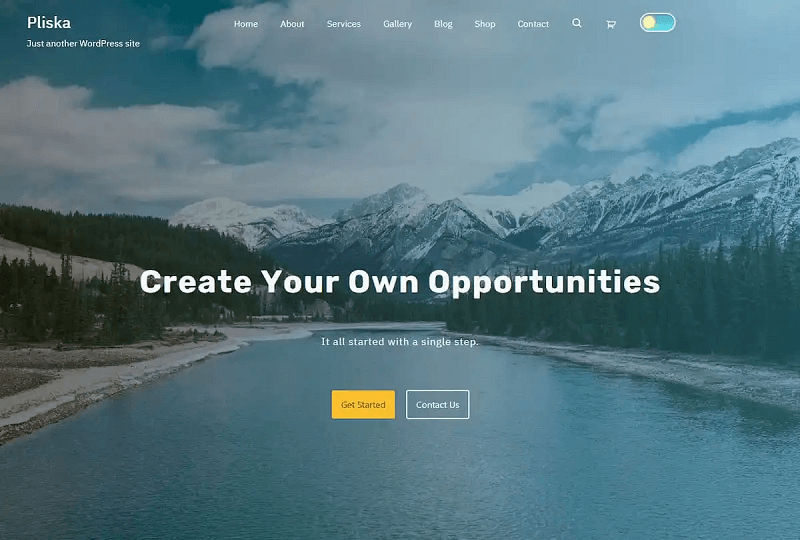**Screenshot from the Pliska Website**

In the top left corner of the webpage, the Pliska logo is prominently displayed. Beneath the logo, a tagline reads, "Just another WordPress site." On the same row, a navigation menu includes tabs labeled: Home, About, Services, Gallery, Blog, Shop, and Contact. Accompanying the menu are a search button, a shop button, and a toggle button. 

The background wallpaper features a stunning mountaintop covered in snow, with a serene river flowing at its base. The river is bordered by dense clusters of pine trees, suggesting a setting in either the Pacific Northwest or a cold climate region in Europe or North America.

Centrally positioned on the webpage, bold white text proclaims, "Create Your Own Opportunities." Below this title, smaller text adds, "It all started with a single step." Directly beneath this motivational phrase are two side-by-side buttons: a yellow "Get Started" button on the left, and a transparent button with a white outline labeled "Contact Us" on the right.